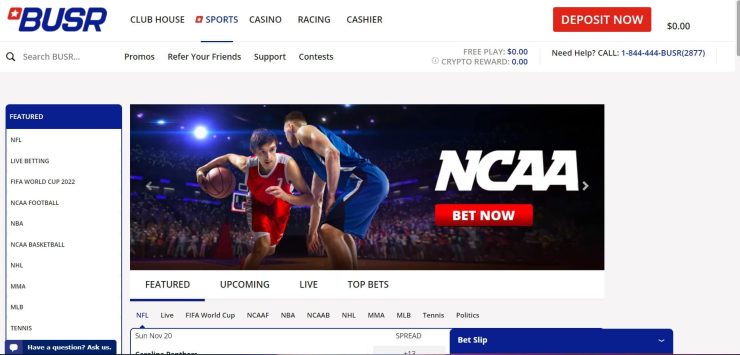Here is a cleaned up and detailed caption for the provided image:

"This image is a cropped screenshot of a BUSR betting website, displayed in a desktop view, characterized by its wide layout. At the top left corner, the BUSR logo is prominently featured. To the right of the logo, the navigation menu includes links labeled 'Clubhouse,' 'Sports,' 'Casino,' 'Racing,' and 'Cashier.' Further to the right, a large red button prominently states 'Deposit Now,' with a displayed balance of $0 adjacent to it. Beneath this section, on the bottom left, there is a search bar positioned underneath the logo. To its right, quick access links for 'Promos,' 'Refer Your Friends,' 'Support,' and 'Contacts' are displayed. To the right side, 'Free Play' and 'Crypto Reward' both show a balance of $0. On the far right, a 'Need Help' section includes a prompt to call customer service with the relevant phone number provided.

The main body of the webpage has an off-white background. A left-hand panel titled 'Featured' at the top, highlighted in a blue box, lists various betting categories: NFL, Live Betting, FIFA World Cup 2022, NCAA Football, NBA, NCAA Basketball, NHL, MMA, MLB, and Tennis. At the bottom of the panel, it states 'Have a Question, Ask Us,' with the remainder of the content cut off in the screenshot."